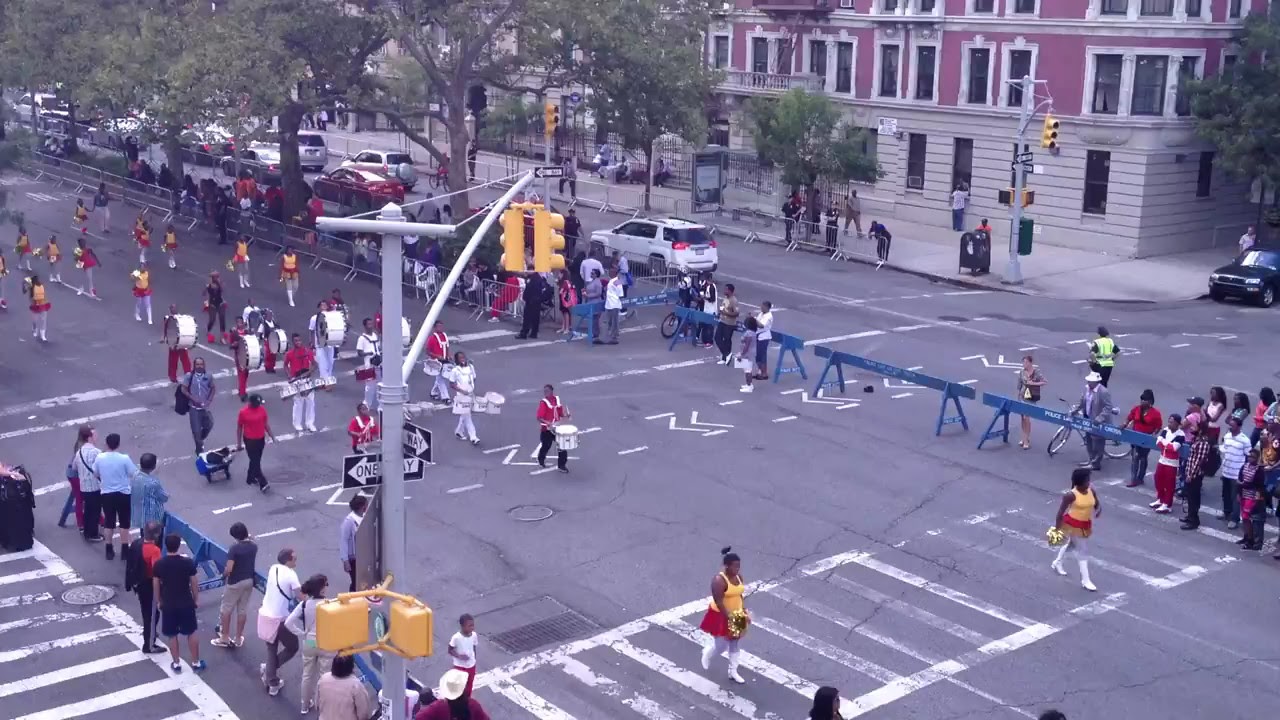The image depicts a vibrant and bustling parade winding through a large city street, characterized by its wide lanes and urban setting. The street, marked with crosswalks and barricades on either side, is filled with a lively crowd of onlookers enthusiastically watching the procession. At the forefront of the parade are cheerleaders in striking red and yellow uniforms, complete with white boots and gold pom-poms, standing confidently at the crosswalk. Following closely behind is a dynamic marching band, composed of predominantly black high school students, featuring drummers and band members in coordinated red attire carrying various instruments. The parade proceeds from the top left towards the bottom right corner of the image, navigating a street marked by stoplights and colonial-style buildings. Cars are parked along the roadside, and green trees add a splash of nature to the scene. The midday sunlight bathes the entire setting, highlighting the colorful spectrum of white, grey, yellow, red, light blue, and black along the street and in the attire of the participants.